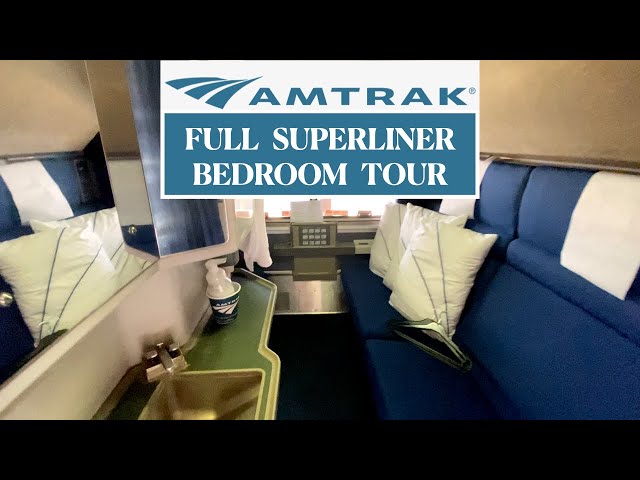The image depicts a narrow, high-end train compartment that resembles a compact hotel room and is likely a thumbnail for a video, given the black horizontal bars on the top and bottom. At the very top center of the image, a white rectangle contains the Amtrak logo, which consists of three slightly twisted bars, and the word “Amtrak” in blue letters. Below this, a blue rectangle features the phrase “Full Superliner Bedroom Tour” in white text. 

Inside the train compartment, the right side features a blue sofa adorned with white pillows and accompanied by a few coat hangers. The left side showcases a green countertop with a metal sink, a blue Amtrak cup, and a soap dispenser. Above the countertop is a white wall topped with a large mirror. The back of the compartment includes a window and a gray panel with buttons, likely serving a functional purpose within the room. The walls are cream-colored, contributing to the luxurious and cozy ambiance of the space.